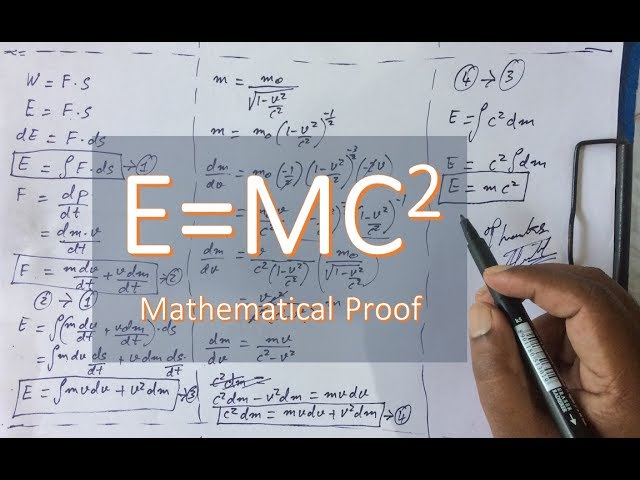In this image, we see a white sheet of paper with mathematical equations written in black ink, divided into three vertical sections separated by dotted lines. The final formula on the paper is Einstein's famous equation, E=mc². At the bottom right of the paper, a dark-skinned hand is holding a black pen. The image has been edited to include text in the middle, reading "E=mc² Mathematical Proof" in white and orange colors. The photo is letterboxed with black rectangular strips at the top and bottom, giving it a screenshot-like appearance.